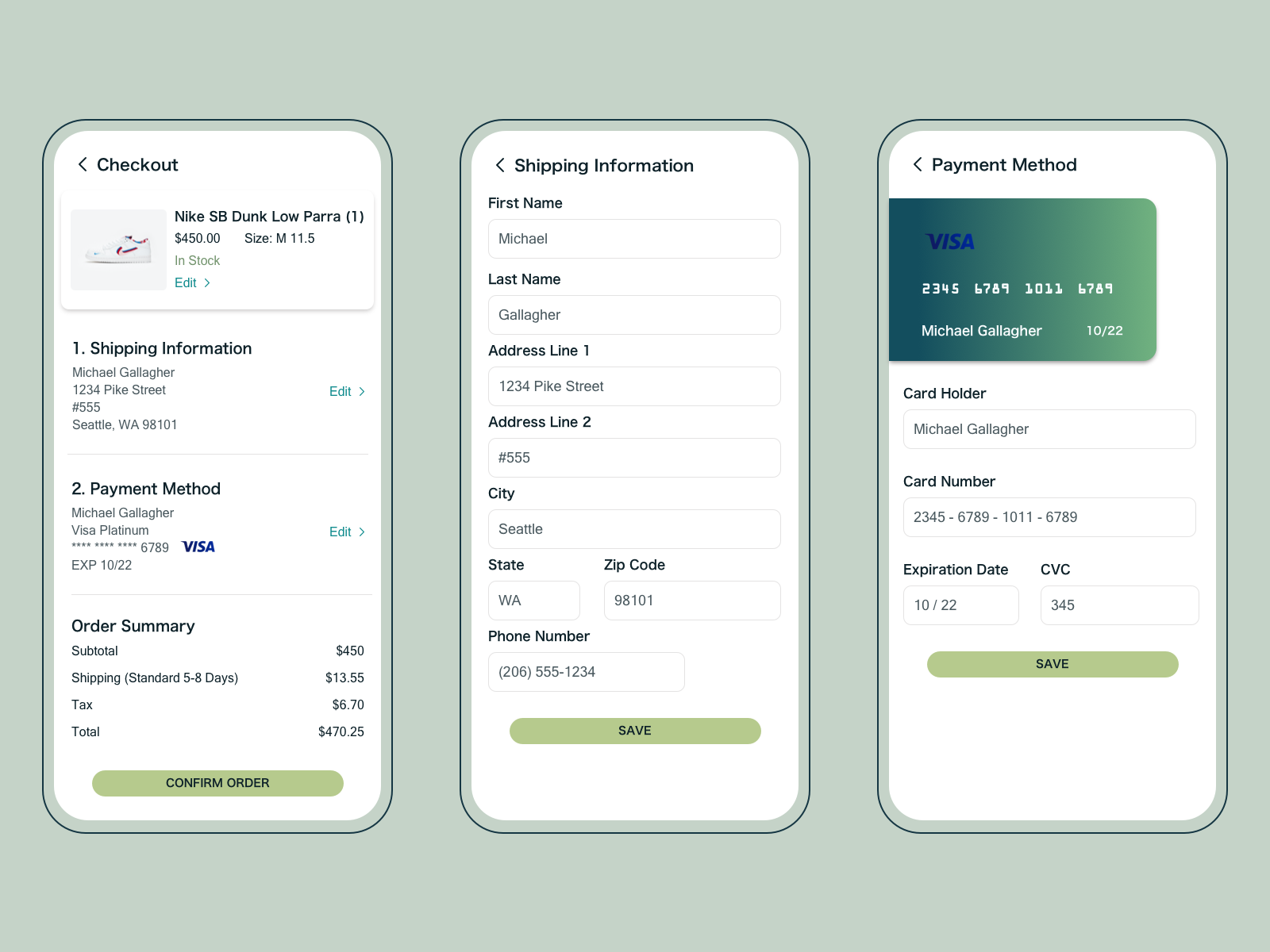The image consists of three detailed screenshots showcasing the online shopping experience on the Nike store website. 

In the first screenshot, the interface displays several essential sections: a prominent "Checkout" button at the top, followed by a detailed view of the selected item—a sneaker labeled "Nike SB Dunk Low." The price is listed as $450. The page also includes different checkout elements such as "Shipping Information," "Payment Method," and "Order Summary" with line items for subtotal, standard shipping (noted as eight days), taxes, and the final total.

The second screenshot focuses on the "Shipping Information" section, where required fields for customer details are presented. It includes spaces to enter "First Name," "Last Name," "Address Line 1," "Address Line 2," "City," "State," "ZIP Code," and "Phone Number."

The third and final screenshot displays the "Payment Method" section. The icon of a Visa card is shown, along with fields to input the "Card Holder" name, "Card Number," and "Expiration Date."

Overall, the images provide a comprehensive view of the steps involved in completing a purchase on the Nike online store.